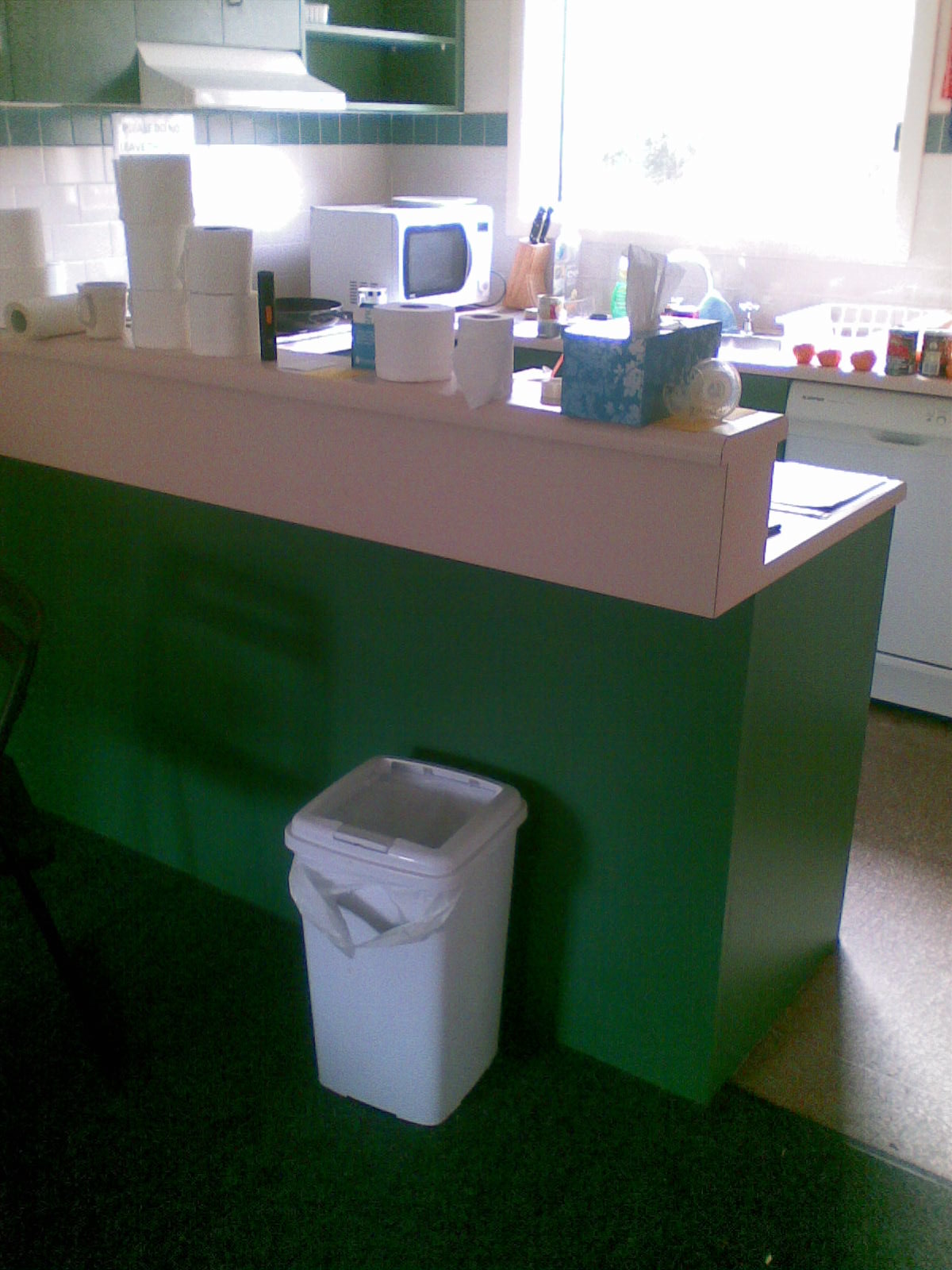A detailed view of a kitchen taken from the adjoining dining area. Dominating the foreground is a white trash can with a conspicuously visible white trash bag. The floor beneath appears to be covered in green linoleum. Partially visible on the left side is the leg and part of the seat of a chair, along with the shadow cast by another chair on the bar that separates the dining room from the kitchen. The bottom half of the bar is painted green, while the top is white. Atop the bar's upper shelf are several rolls of toilet tissue and a box of Kleenex. Beyond this, a microwave can be seen, set against a white tile wall adorned with a green tile border. Further into the kitchen, a knife rack holds a couple of black-handled knives. A sink is positioned beneath a window, and next to it, three ripe tomatoes are on display. Nearby, what seems to be a dishwasher and a dish drainer are situated, with a bottle of dishwashing liquid visible behind the sink.